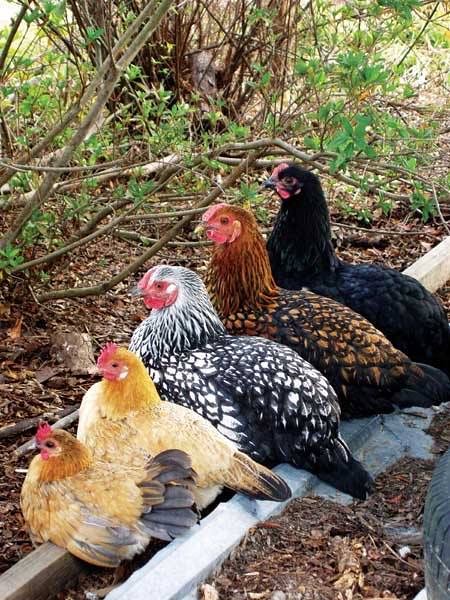The image captures five chickens perched on a wooden beam in an outdoor setting, arranged in a diagonal line from smallest to largest. The scene depicts a forested area with a ground covered in brown leaves and dirt, along with some sparse green leaves on nearby branches. The background includes trees with both green leaves and fallen brown branches. The chickens, all facing left, are distinguished by a range of feather colors and facial markings. The smallest chicken at the lower left has golden brown feathers, a red face, and fluffed-up tail feathers. Following it, the second chicken, slightly larger, also has golden brown feathers, a red face, and a few black tail feathers. The middle chicken features black and white feathering, with a predominant white head and red facial markings. The next chicken in line is even larger, showcasing alternating black and brown colors with a predominantly brown face. The largest chicken at the upper right is mostly black with red on its face. The chickens are seated on two wooden rails, one painted white and the other a natural brown, adding to the rustic feel of the scene.